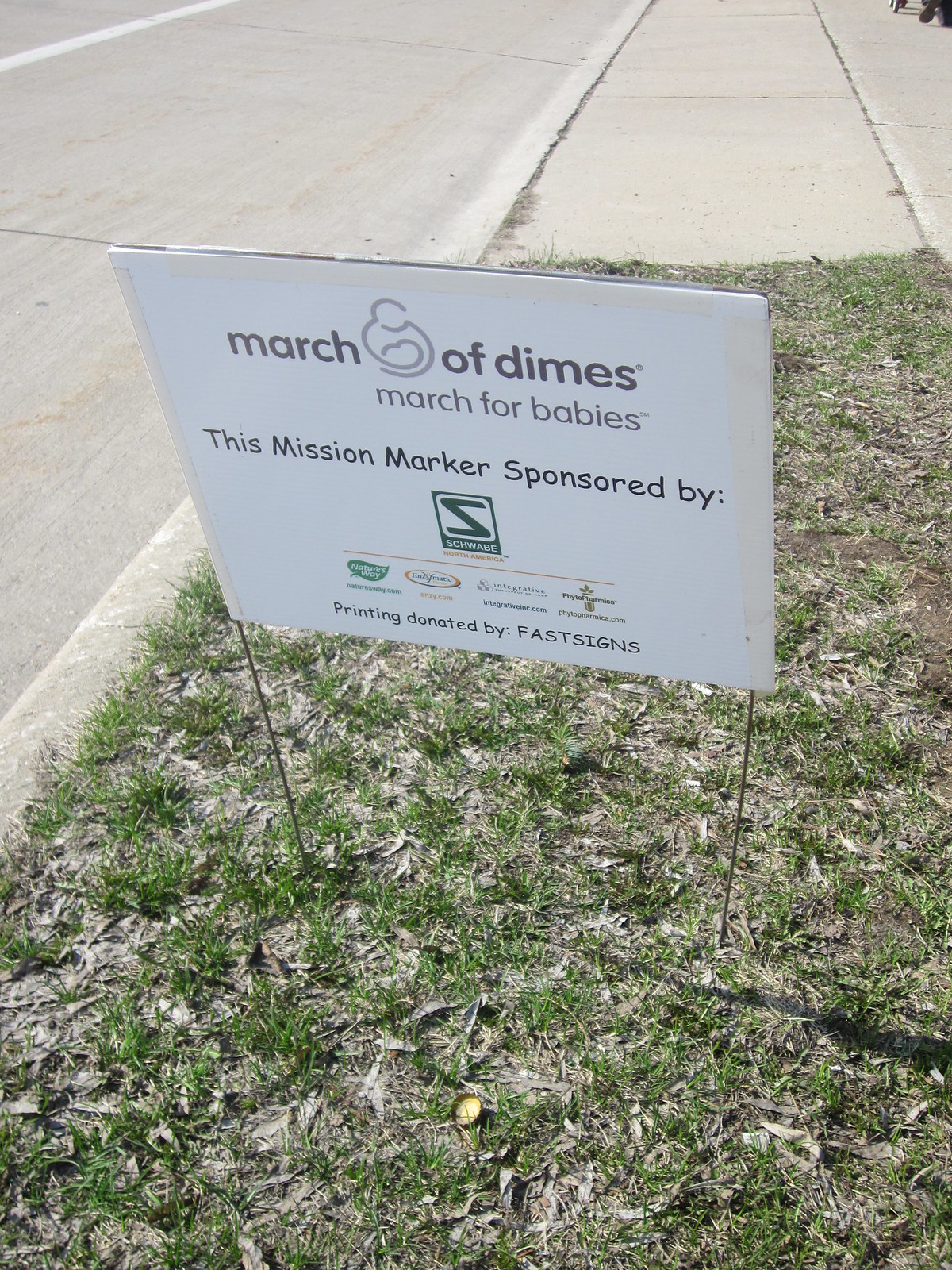In this vertically aligned rectangular image, the focal point is a small outdoor advertising sign situated in a patch of dry, half-dead grass near a sidewalk and street curb. The sign is supported by two thin metal poles. The sign prominently displays the text "March of Dimes, March for Babies," with a likely illustration of a mother holding a child between the words "March" and "of." Below that, it reads, "This mission marker sponsored by," followed by a series of sponsor logos. The sponsors listed are Schwab, Schraube North America, Nature's Way (naturesway.com), Enzymatic (enzy.com), Integrative (integrativeink.com), and Phytopharmaca (phytopharmaca.com). At the bottom, it states, "Printing donated by Fast Signs." The top of the image reveals a sidewalk, and the left side shows a road with a visible white line demarcating two lanes. The color palette includes shades of gray, white, tan, black, green, yellow, and orange. The scene is captured from the perspective of someone standing near the sign, likely in the middle of the day, with the street positioned towards the top left of the image and the sidewalk visible in the background.